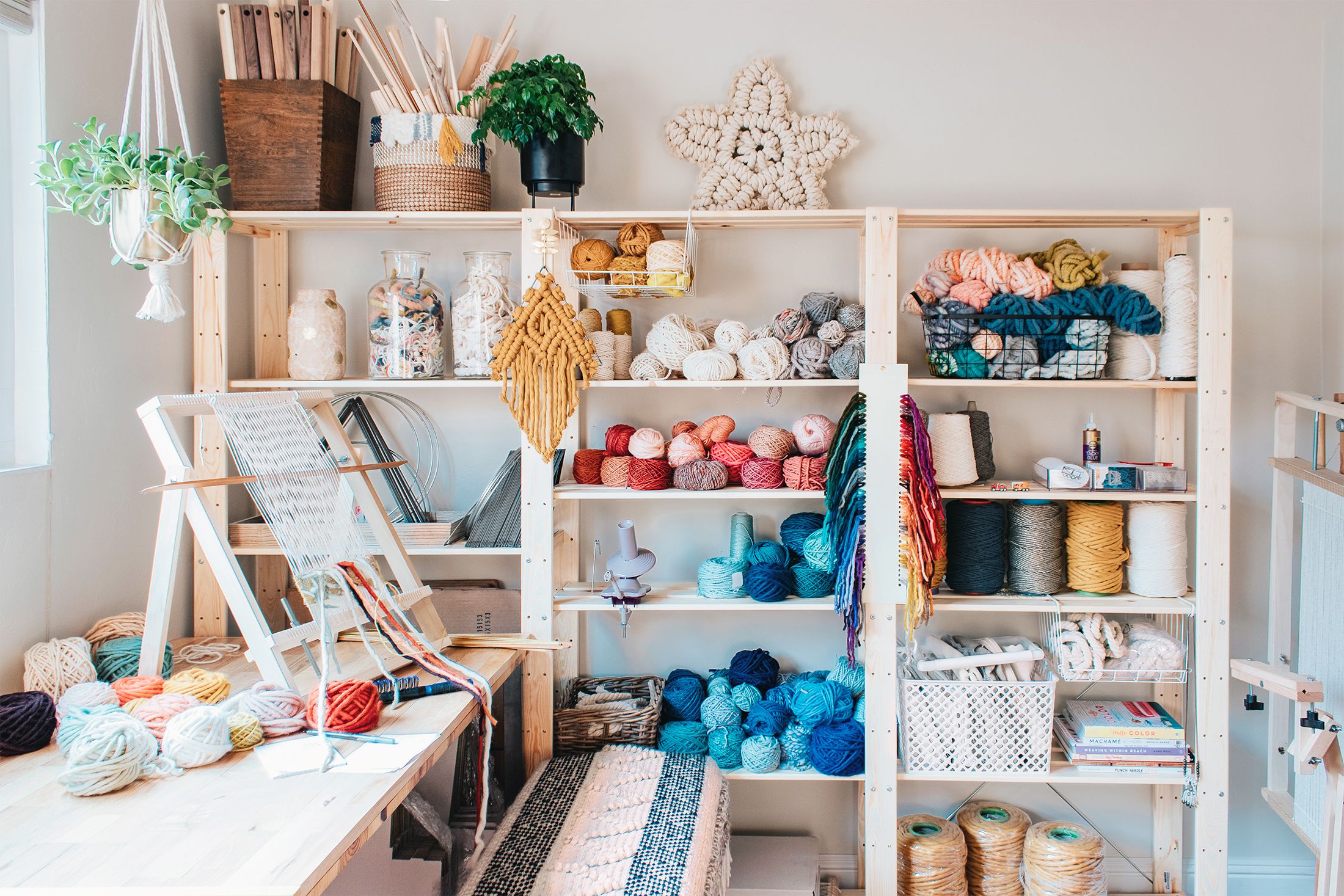The photograph, presented in landscape orientation, captures a detailed view of an interior craft or knitting room with a light gray wall as the backdrop. Dominating the scene is a tall, white wooden shelf structured into three vertical rectangular units. These units vary in the placement of their horizontal boards, creating a dynamic display space. The shelf is laden with numerous balls of yarn in a rainbow of colors including white, red, dark red, blue, light blue, brown, and gray, alongside several jars and baskets filled with yarn and spools. Crowning the shelf is a macrame star made of white yarn, subtly emphasized by a small plant with greenery placed nearby. 

In the left foreground, a wooden table is visible, accompanied by a bench adorned with a pink and blue striped blanket. Atop the table sits a weaver's loom, its pine frame supporting white threads intertwined with a shuttle and additional yarn strands. To the left, the scene captures a plant hanger and a small straw basket adjacent to a window opening. All these elements, with a photographic realism style, create an inviting and meticulously organized space dedicated to crafting and knitting activities.